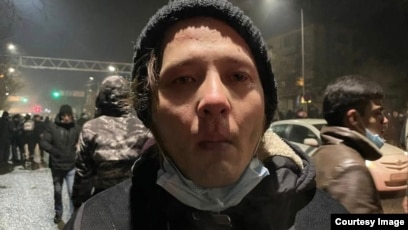In this detailed winter scene, a rectangular image showcases a nighttime city setting amidst a probable protest or traffic standstill. The stark, cold atmosphere is palpable with numerous people bundled up in thick jackets and beanies, indicating the wintery conditions. Central to the image is a person with light skin wearing a black hat and a zipped-up black coat. This individual, looking directly at the camera with a sorrowful expression and possible tears, has a face mask pulled down to their chin. In the background, tall buildings loom under the black sky, illuminated by a green traffic light. To the right, a yellow car is visible, and another person with a brown jacket and mask similarly pulled down is seen looking to the right. The scene also features what appears to be a metallic barrier, possibly railway-related, hinting at a complex urban environment. The bottom of the image bears the text "courtesy image," suggesting it was taken by a journalist.